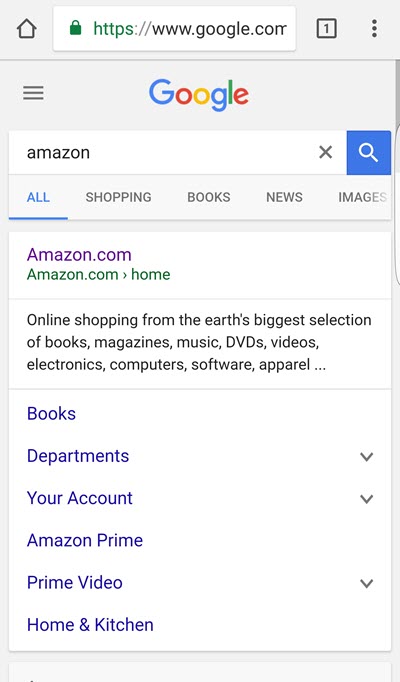This image captures a screenshot from a website with a light grey background. At the top, there is a minimalist outline of a house, followed by a white address bar featuring a green padlock icon with "HTTPS" in green text, and the website URL, "www.google.com", displayed in black. Adjacent to the address bar, there is a black outline with the number "1" inside, alongside three vertically aligned dots.

Below the address bar, the background remains grey, and three horizontal lines are displayed on the left side. Centrally positioned, the word "Google" is prominently featured in its classic logo style, with the "G" in blue, the first "o" in red, the second "o" in yellow, the second "g" in blue, the "l" in green, and the "e" in red.

Continuing downward, there is a white search bar displaying the text "Amazon." To the right of this search bar, an "X" is present for clearing the text, followed by a blue square containing a white magnifying glass icon.

Below the search bar, navigational options are listed: "All," "Shopping," "Books," "News," and "Images," where "All" is highlighted in blue text with a blue underline.

Further down, the content displays a white box with "Amazon.com" in purple print, followed by another instance of "Amazon.com" with an arrow pointing to "Home." Below this, there is a brief description of online shopping and various options listed: "Books," "Departments," "Your Account," "Amazon Prime," "Prime Video," and "Home and Kitchen."